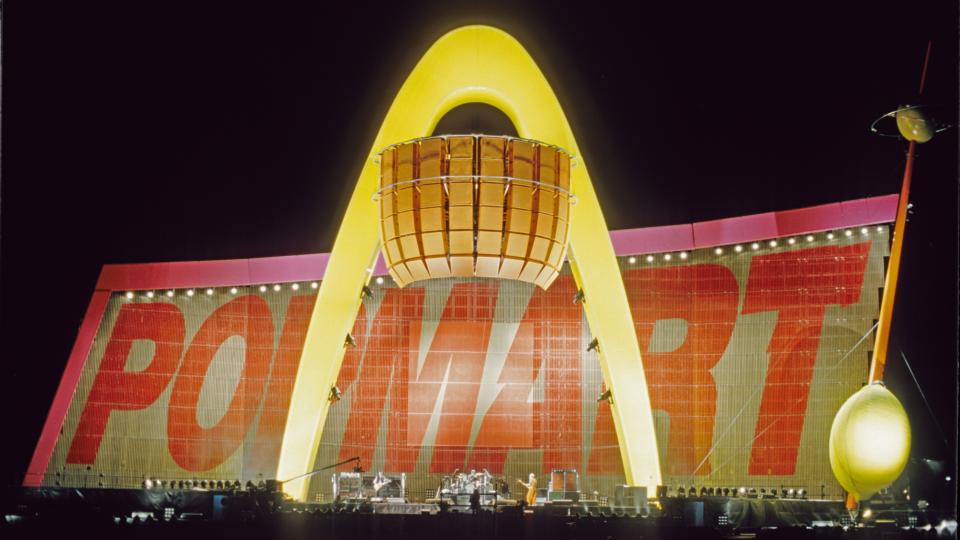The image depicts an outdoor nighttime concert at a large music festival, evidenced by a towering backdrop and a sizable audience. Dominating the scene is a significant banner with the words "Pop Mart" boldly written in red letters, bordered by pink. The banner is so immense that the band performing on stage, equipped with musical instruments like a drum kit and a guitar, appears diminutive in comparison. Above the stage arches a striking, modern-looking yellow arch, reminiscent of a sci-fi design. The arch seems to incorporate an oval element with a gold rod, possibly resembling an abstract planet with a moon orbiting it, adding a fantasy or futuristic touch to the scene. Stage lights, shadows, and silhouettes of the heads of concertgoers are visible against the stark black nighttime sky, enhancing the dramatic ambiance.